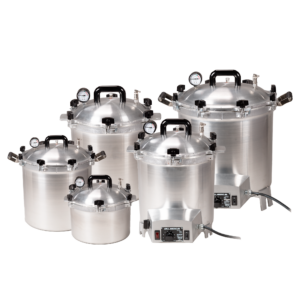This is a detailed image of five stainless steel pressure cookers, arranged against a stark white background. They vary in size, ranging from one comparable to a common cooking pot used in a typical home to larger, more industrial-looking models. Each pressure cooker is equipped with thick black handles on the sides and lid, as well as black knobs and a pressure gauge on top. 

The smallest cooker sits to the left, resembling a pot used for boiling pasta. Slightly behind and to the right is the second smallest cooker, taller and wider than the first. The next in size is partially obscured by the second cooker but notably larger. The second largest cooker is partially hidden behind the previous ones, with the largest unit prominently displayed on the far right. All the cookers are made of shiny stainless steel, reflecting the light, and the largest two feature units with black cords for plugging in, indicating they may also have electric components.